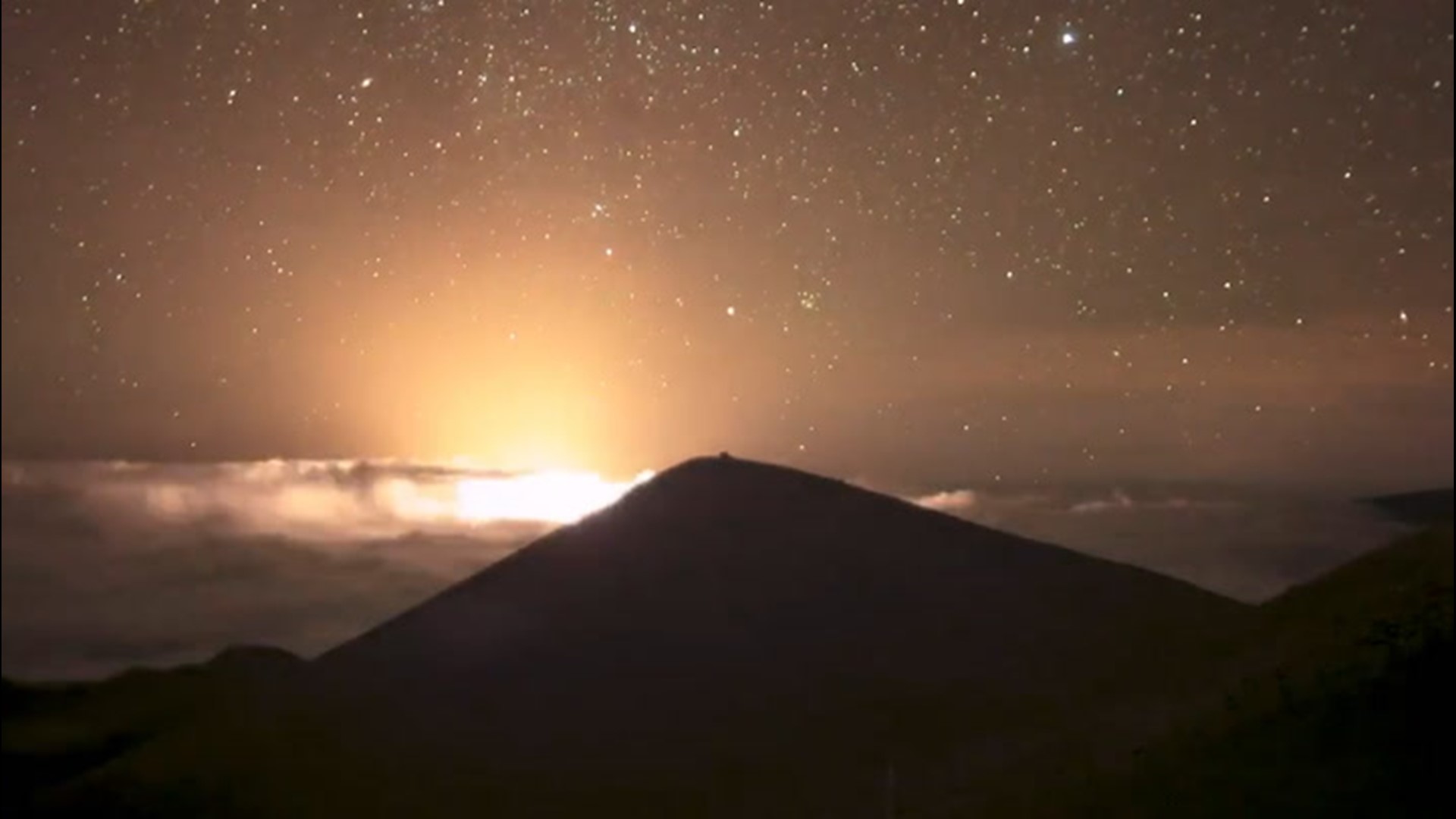This captivating landscape photograph, taken from an elevated position, showcases a serene and dramatic nighttime scene. Dominating the center is a prominent hill with a peaked top, silhouetted against a large, shimmering body of water that stretches beneath it. The water, animated with gentle waves, reflects a rich orange hue, a striking attribute that permeates the entire image. Just beyond this large body of water, a brilliantly radiant light, presumably the setting sun, bathes the horizon in its warm glow, partially veiled by wisps of clouds. The sky above is a deep night canvas dotted with countless twinkling stars, lending a magical quality to the scene. In the bottom right corner, dark spiky formations jut from the ground, adding texture and contrast to the composition. The collective elements—vivid colors, striking silhouettes, and a profusion of stars—harmonize to produce a mesmerizing and tranquil image.